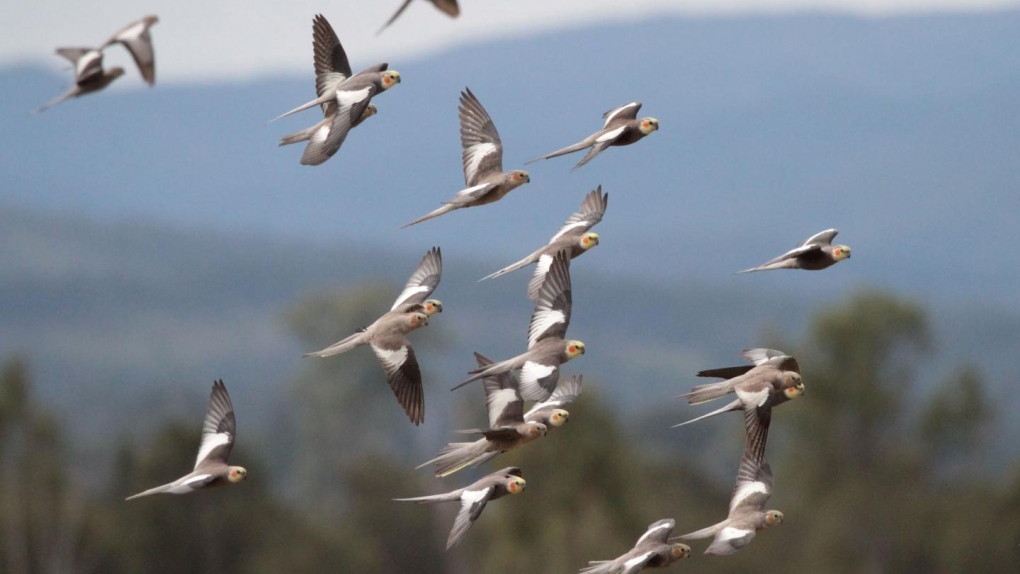In this detailed photographic image, a disorganized flock of approximately 17 to 20 birds, likely doves or parrots, is captured mid-flight against a muted, blurred background. The sky forms the upper portion of the backdrop with soft blues and hints of white clouds, while the lower half reveals the distant tree line and vegetation. The birds, which are in sharp focus, display a mix of gray and white plumage with distinctive markings: white areas close to the body, gray and black wingtips, orange-red spots near their eyes, and a hint of yellow on their necks. Their bellies appear black, possibly accentuated by the shadow of the sun from behind. The birds are all flying from left to right in a somewhat scattered, non-V formation, showcasing various stages of wing flapping with their tail feathers prominently gray and white.